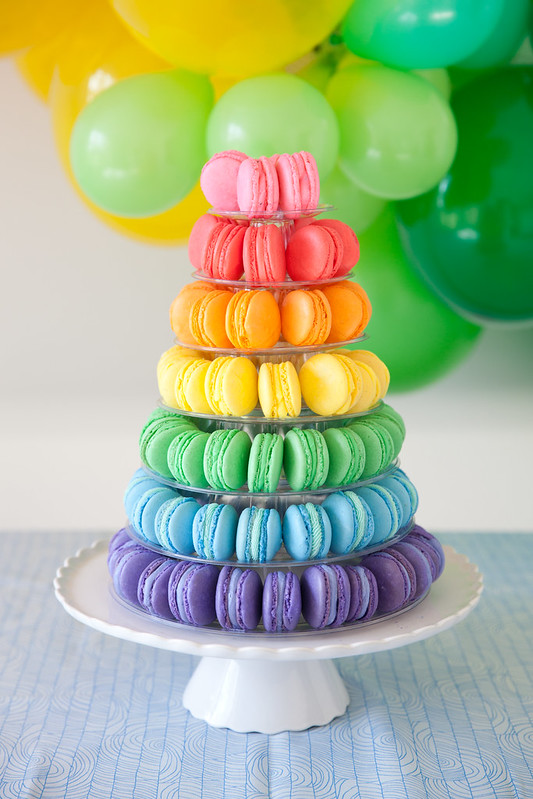The image showcases a meticulously arranged tower of colorful macarons on a large, white pedestaled cake plate. The macarons are organized in seven tiers forming a cone-like structure, starting from the bottom with purple, followed by blue, green, yellow, orange, hot pink, and finishing with pale pink macarons at the very top. Each macaron is displayed horizontally, revealing both sides of the cookie and the creamy filling inside. This elegant display sits atop a table draped with a white and blue tablecloth featuring a swirled design. In the background, festively colored green, yellow, and blue balloons float against a white wall, enhancing the celebratory atmosphere.